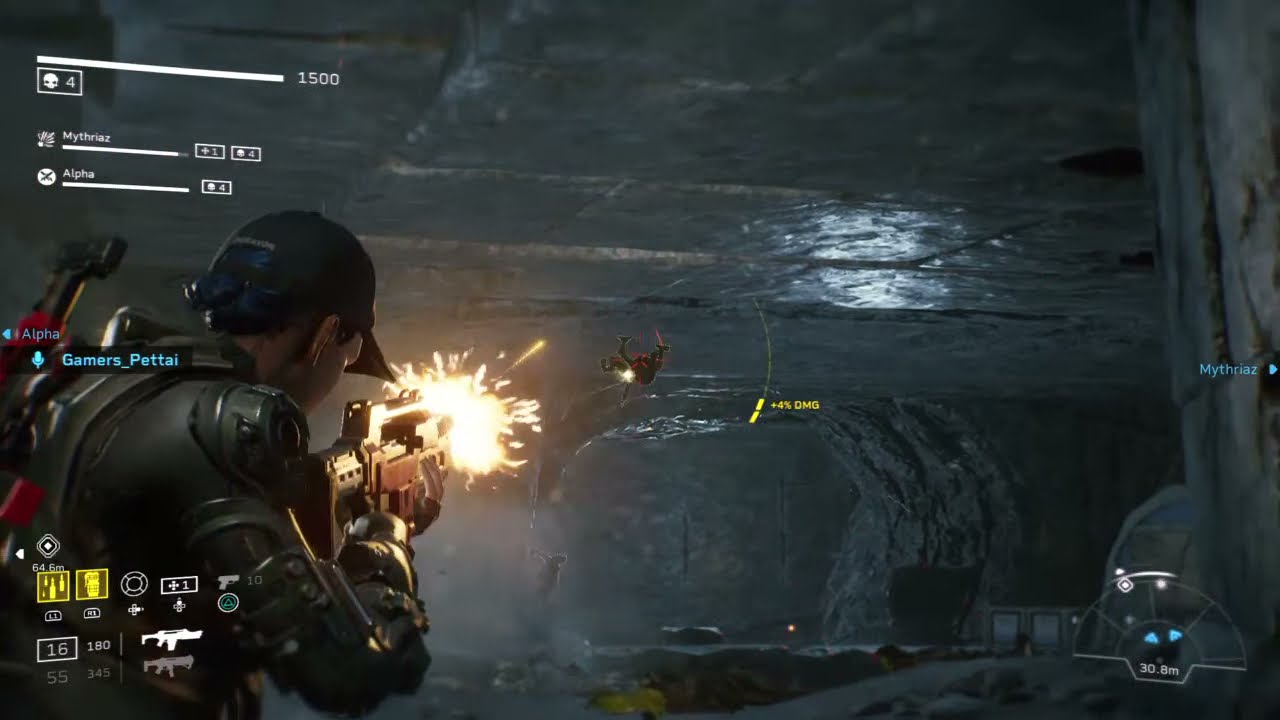This screenshot from a shooting video game captures an intense moment set in a vast, gray, cave-like structure. The central character, positioned on the left side of the screen, is equipped with high-tech black armor and a black baseball cap, with black hair tied back in a bun. The character is firing an automatic weapon, vividly represented by yellow sparks and flames emanating from the gun's barrel. Mid-frame, an alien creature appears to be hit by the gunfire and is flying backward, with chains noticeable around it. The game's interface displays various icons and stats: Player names 'Myalthros' and 'Alpha' with a score of 1500 are visible, along with health bars at the top, a chat in the center left, weapon selection in the bottom left, and a mini-map in the bottom right corner.